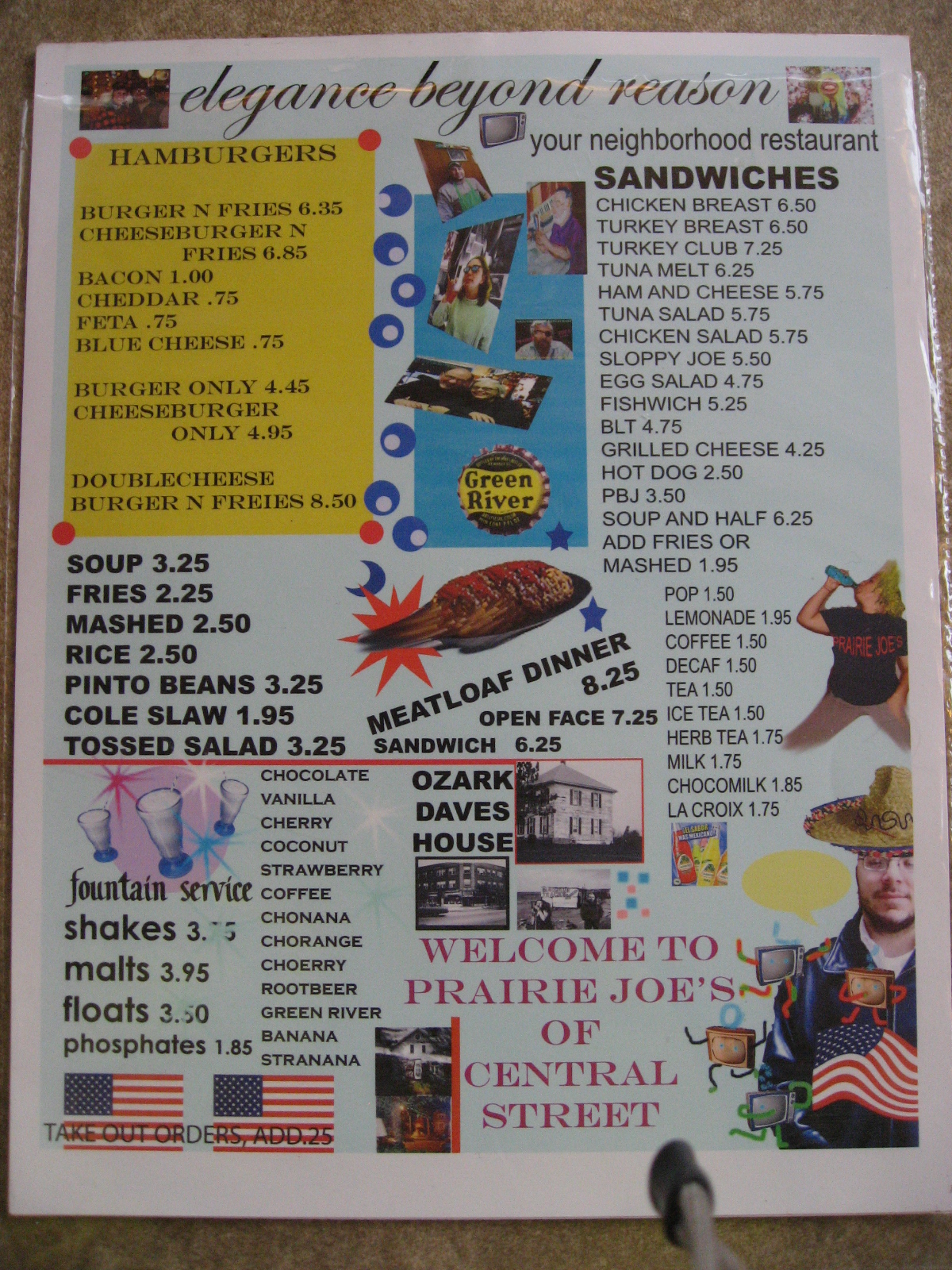This laminated menu from a restaurant is designed with a nostalgic, old-style café aesthetic, featuring a blend of vibrant colors and inviting imagery. At the top, the menu proudly proclaims "Elegance Beyond Reason - Your Neighborhood Restaurant," setting a welcoming tone. Below this, there's an extensive list of sandwiches, accompanied by offerings like meatloaf, soup, fries, mashed rice, and pinto beans. The menu also includes a dedicated hamburger section and a fountain service.

The bottom of the menu presents two American flags, symbolizing a patriotic touch, next to the note “Take Out Orders Welcome.” Highlighting the local charm, it warmly invites patrons with “Welcome to Prairie Joe’s of Central Street” in striking magenta text, contrasting against the predominantly black typography used throughout.

In the lower right corner, an image of a man in a cowboy hat or sombrero adds a whimsical touch. The overall color scheme transitions from yellow and blue to light blue backgrounds, complementing the classic diner look reinforced by the laminated finish typical of southern cafés. The prices for all the items are clearly listed, ensuring a straightforward dining experience.